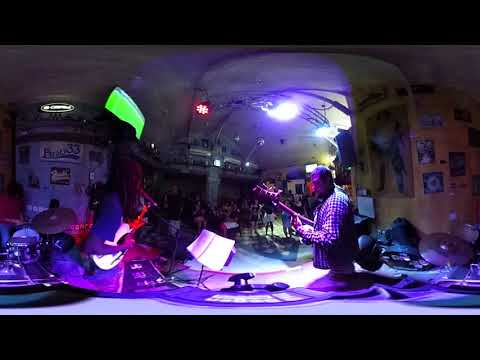In the image, a dimly lit bar or small concert hall serves as the backdrop, illuminated primarily by purple lights. The panoramic photo captures a live music performance, centering on a man in a plaid shirt playing guitar. To his left stands another guitarist, who also appears to be singing, and further left is the drummer, partially obscured by cymbals and the drum set. The ambiance is intensified by the neon lights from bar signs scattered around the room.

The scene appears to be viewed from the stage amidst the band members, offering a unique perspective where the audience and dance floor are visible in the background. A small crowd watches the band, creating an intimate setting typical of a house band performance. On the left side of the image, a TV mounted near the ceiling shows what looks to be a football match, adding to the bar's lively atmosphere. The walls are a mix of blue and wooden panels adorned with beer signs, and the ceiling is brownish and relatively high. This visual detail enhances the cozy and immersive nighttime experience of this music bar.